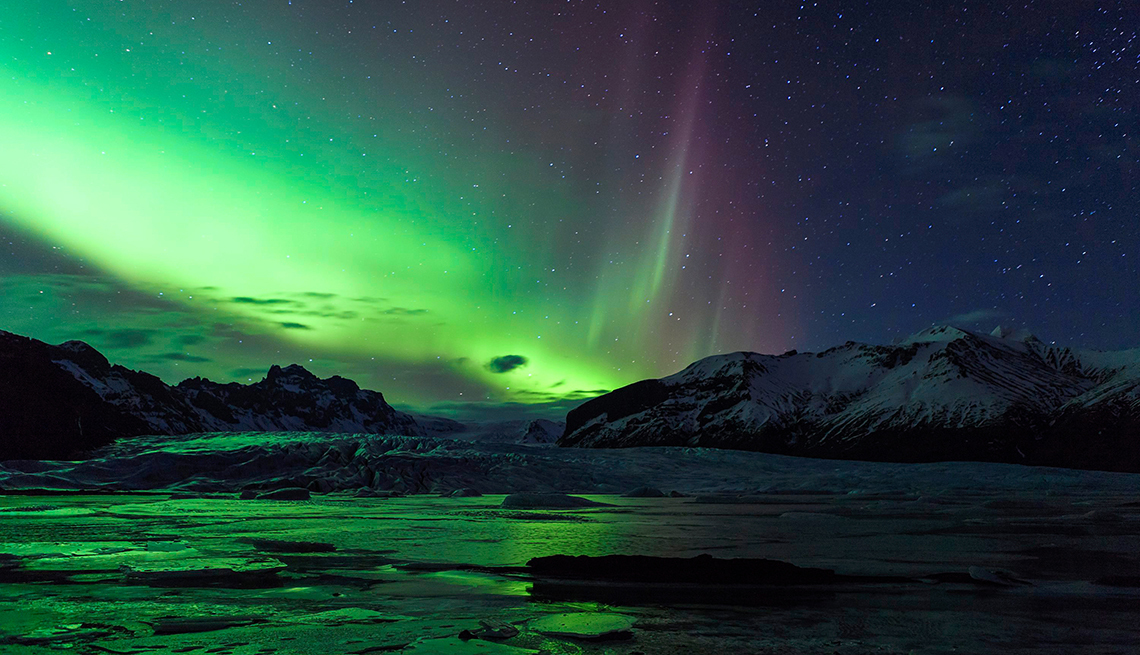This professionally taken image captures the stunning Northern Lights in a dark nighttime outdoor setting, possibly in Alaska. The photo showcases a wide landscape with prominent snow-covered mountains on both sides—the ones on the right being larger and more prominent. A serene lake with scattered pieces of ice lies at the base of these mountains. The sky above, adorned with stars primarily on the right side, glows vibrantly with shades of neon green fading into purple, emanating from the Northern Lights. This mesmerizing display of green and purplish hues reflects vividly on the lake and the icy surface, creating a breathtaking and ethereal atmosphere. Dark clouds are also visible amidst these vivid lights, adding depth to the scene. The overall color scheme is dark, emphasizing the luminance of the Northern Lights against the night sky.